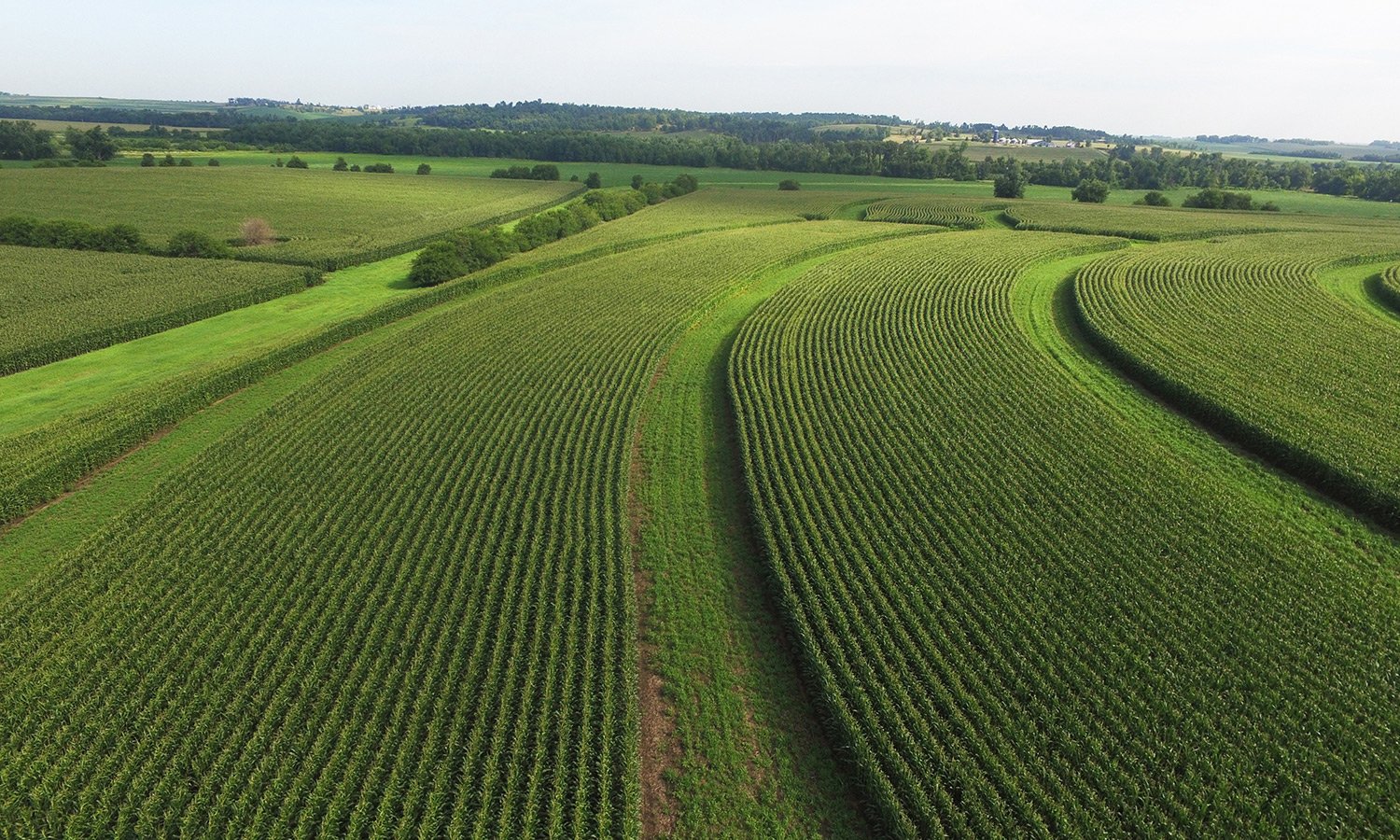This aerial photograph captures a vast rural field, likely used for farming, with a clear blue sky overhead. The field is divided into several sections of vegetation, possibly corn or another crop, growing in rows with grassy walking paths between them. There are at least four distinct rows of crops, interspersed with grassy gaps. In the far distance, a cluster of buildings, possibly farmhouses or a small village, is visible, surrounded by trees and rolling hills. The left side of the image features a larger grassy area transitioning into what seems like more uniformly planted crops. No people, vehicles, or text are present in the image. The scene is predominantly green with shades of white and blue, and hints of dirt in the foreground, suggesting a well-maintained but expansive agricultural landscape.